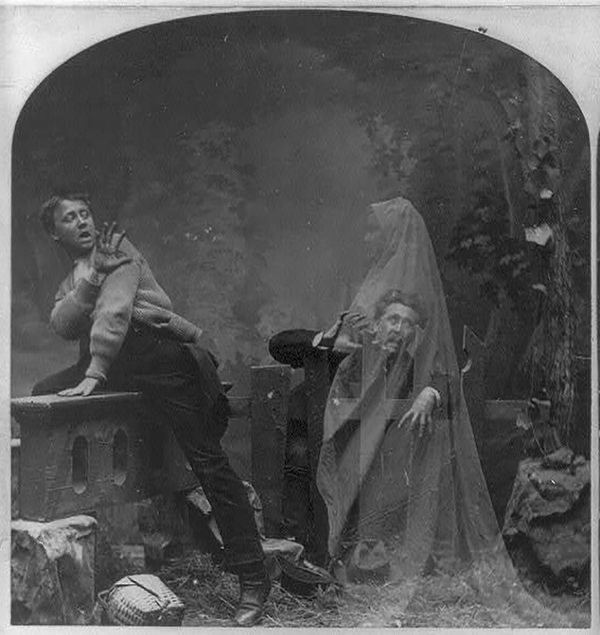The black and white image, whether a photograph or painting, presents a chilling scene. Two terrified men, one younger and mid-leap over a brick fence with one leg over and hand pressing down, the other slightly older and hiding behind the same fence, frantically raise their hands as if to ward off an eerie presence. Both men wear expressions of sheer terror, their mouths agape as they grapple with the fence. Superimposed on the scene is a ghostly figure of a woman, barely discernible through her ethereal veil, standing in front of the older man, who gazes at her in horror. Her spectral form is semi-transparent, adding to the spooky atmosphere. The setting appears to be outdoors, cloaked in darkness, with shadowy vines, trellises, and what looks like a dilapidated building or graveyard, complete with a falling cross in the background. The ground is strewn with indeterminate objects, amplifying the sense of decay and dread.